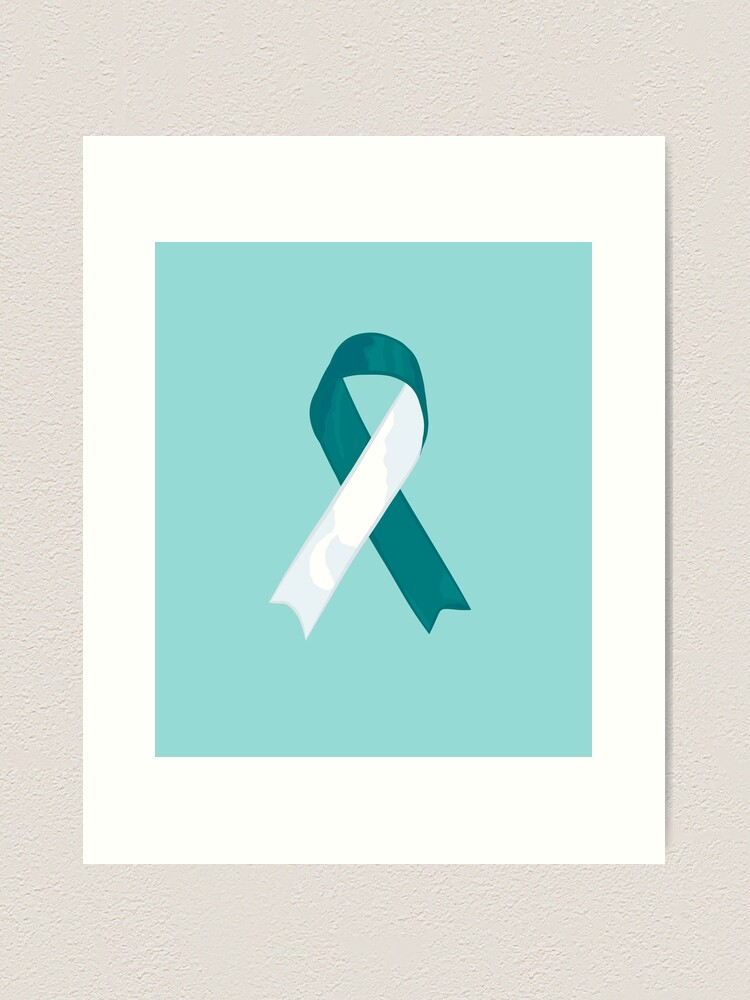The image depicts a digitally created poster hanging against a textured, painted white wall that has a grainy or stucco appearance. The poster itself features a large white rectangular border that frames a central light blue or greenish-blue background. In the middle of this colored background, there's an illustration of a ribbon that is narrow and long, ascending diagonally to the left, curling around, and then descending diagonally to the left again, forming an X shape. The ribbon is primarily black or dark bluish-green on one side with the other side in white, and it incorporates shadows and shading to give it a three-dimensional look. The ribbon's design resembles symbolic awareness ribbons, though its specific meaning is not clear.